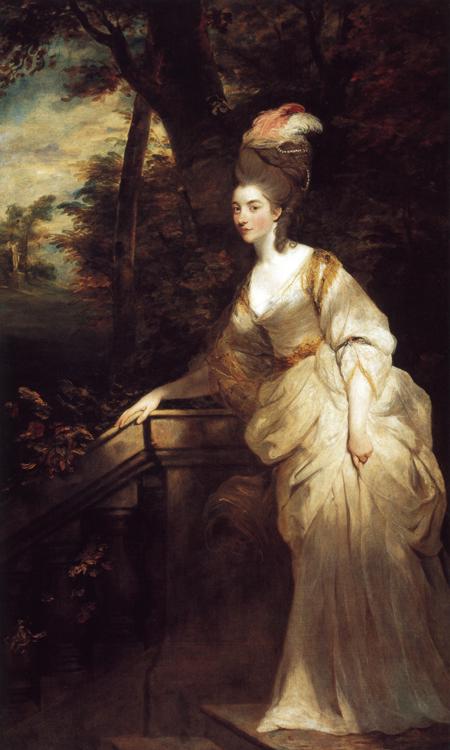This vertical rectangular painting portrays an elegant woman in a luxurious, floor-length, gold-beige dress with abundant draping folds. The dress has three-quarter length sleeves, exposing her lower arms, wrists, and hands. Her gown is squared at the neckline, revealing part of her décolletage. She has high, thick brown hair adorned with an elaborate arrangement of pink and white feathers, adding to her sophisticated appearance. Her face, marked by subtle yet graceful makeup, features a wry smile.

The woman leans with one hand on a grey stone or marble banister, suggesting she is on a grand staircase. The background hints at an outdoor setting with trees and possibly clouds, lit subtly by natural light that casts shadows on her dress. The intricate details of her attire and her poised demeanor suggest she could be a lady of high society or possibly a courtesan from an earlier era.